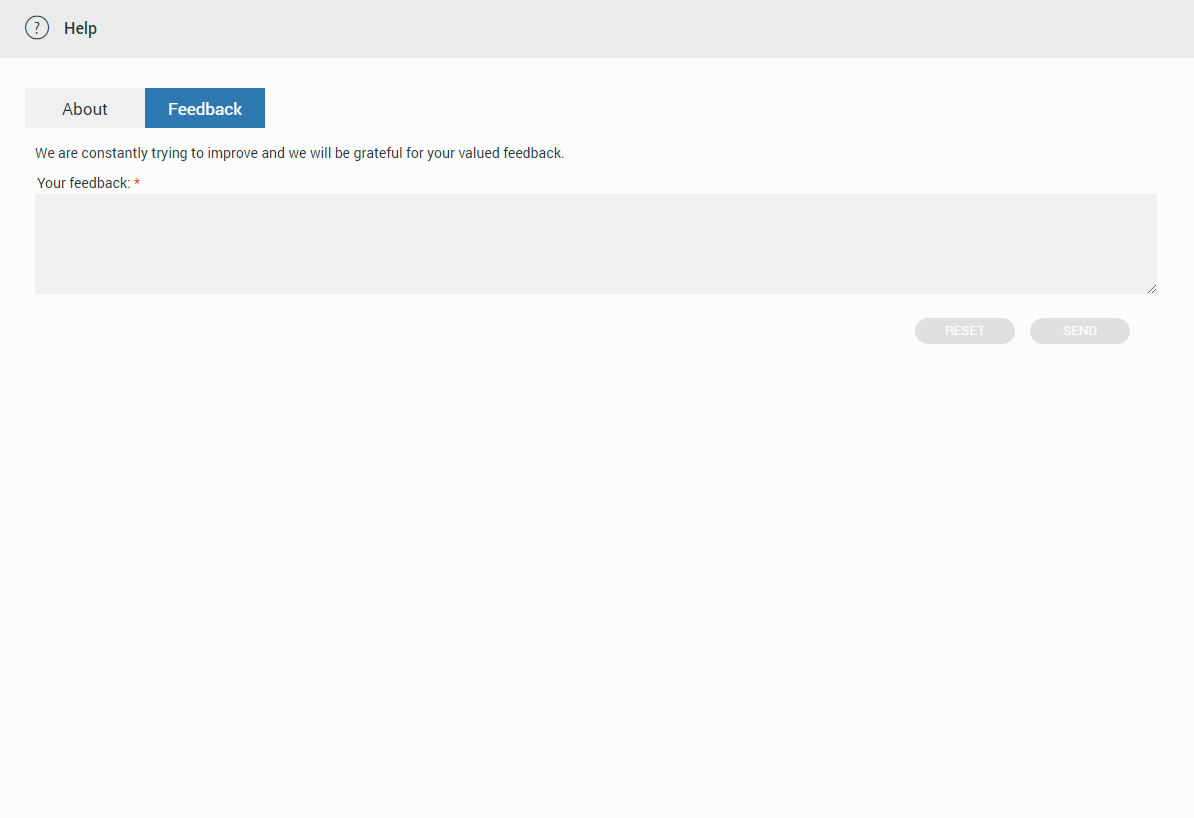This is a detailed screenshot of the feedback section of a webpage. At the very top, there is a light gray bar that spans the width of the screen. On the left side of this bar, a "Help" button appears in gray text, next to a question mark icon enclosed in a circle.

Below this top bar, there is a lighter gray section. On the left side of this section, you see two buttons: "About" in light gray text and "Feedback" in blue text, indicating that the feedback section is currently selected.

Directly beneath these buttons, there's a message that reads, "We're constantly trying to improve and we will be grateful for your valued feedback." 

Following this message, there's a prompt labeled "Your feedback" marked with a red asterisk, signifying that providing feedback is mandatory. Below the prompt, there is a large, darker gray text field where users can enter their feedback.

At the bottom-right corner of this section, there are two pill-shaped buttons: a "Reset" button and a "Send" button, both in gray.